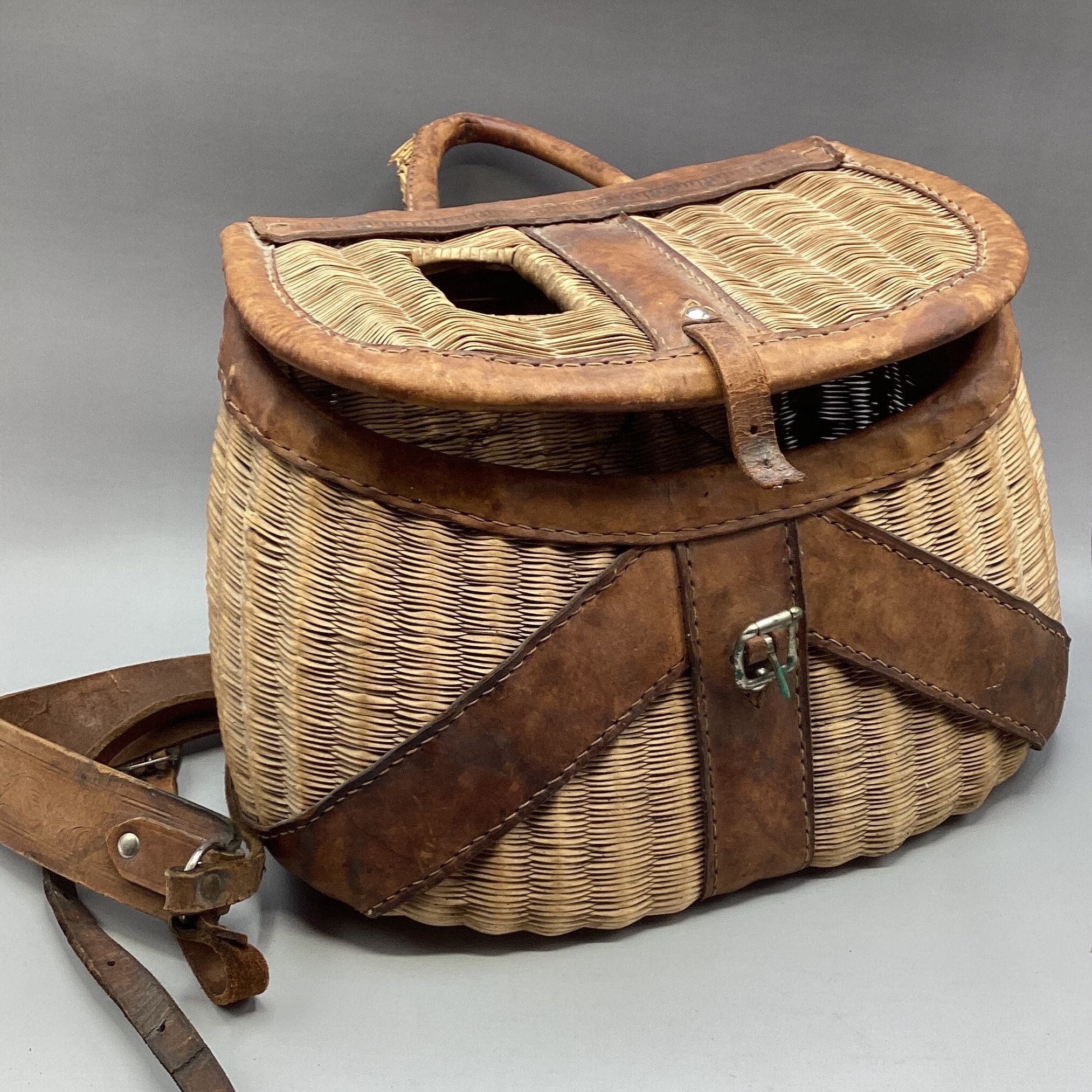This image depicts a detailed, vintage-inspired purse that appears to combine the elements of a basket and woven straw. The main body of the purse is crafted from light brown leather, with intricate weaving reminiscent of traditional wicker baskets, resulting in a textured, tan interior. The bag features a distinctive shape with a rounded rim on one side and a flat edge on the opposite side. A durable handle made from leather extends from one end of the purse, complementing the overall design.

Prominently, there is a central leather strap that secures the lid, which includes a small, square opening on the left side, allowing a glimpse into the dark interior. This strap is notably torn at the end, with two holes visible, indicating wear. Additionally, there is a partially visible belt with a silver-colored rivet towards the bottom left of the purse.

A golden-type buckle adorns the middle of the bag, adding a touch of metallic contrast against the various brown shades. The background is unobtrusive, featuring a gradient of gray tones that range from light at the bottom to dark at the top, ensuring that the purse remains the focal point of the image. The base rests on a lighter gray surface while the upper section fades into a darker gray, enhancing the overall subdued aesthetic of the scene.